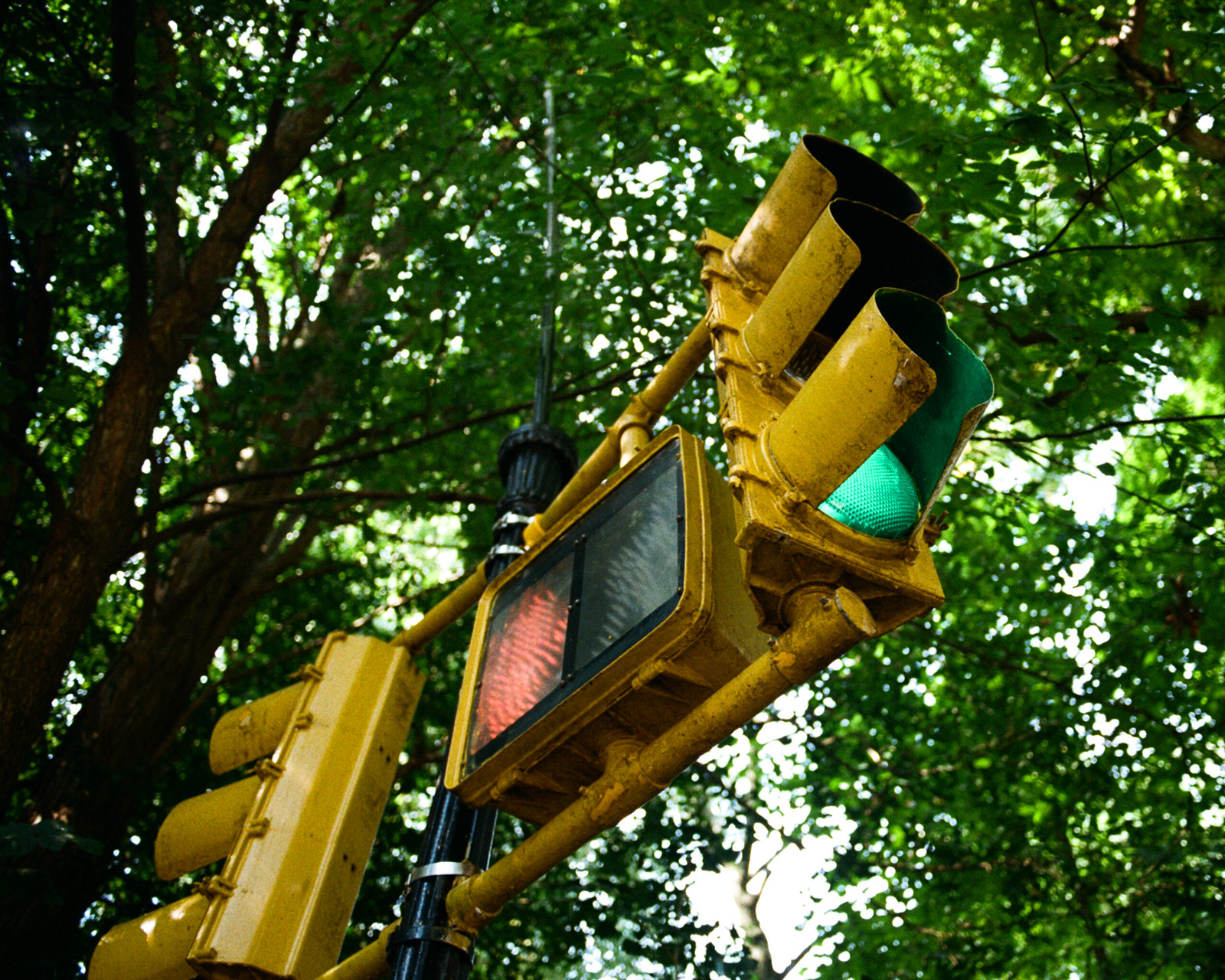This up-view photograph captures a detailed scene featuring two yellow traffic lights mounted on a black pole. The left-hand traffic light is positioned diagonally, while the right-hand one is facing directly towards the right. Between these traffic lights, there is a walk sign illuminated with a red hand, signaling pedestrians to stop. 

Above the traffic lights, the sky appears white, partially obscured by the underneath foliage of silhouetted trees, which are more prominent on the left side and show more green on the right. The traffic light on the right is slightly dirty, but you can clearly see the green light under its metal shade. The traffic lights have a distinctive upside-down U shape due to their half-cylinder design. Overall, the image provides a rich visual of an urban street scene framed against a backdrop of trees and sky.